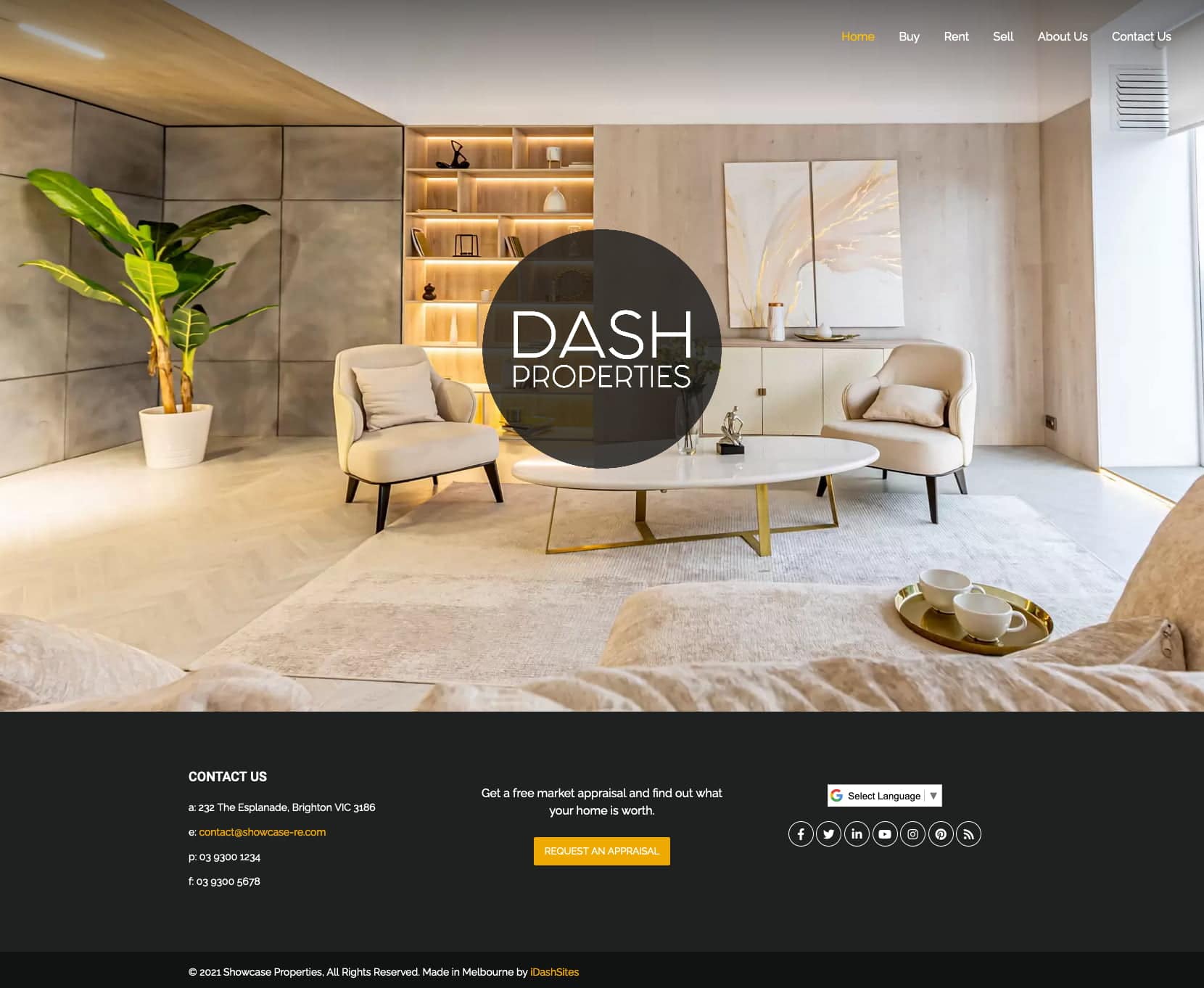Screenshot of a website homepage primarily showcasing a stylish, modern living room. The living room features grey tiled walls contrasting with a pristine white ceiling. A plush white rug adorns the floor, upon which sits a sleek circular coffee table flanked by two puffy white chairs. Dominating the foreground is a luxurious white couch paired with a matching ottoman, topped with a tray holding two teacups. Additional elements include air conditioning vents and a potted palm, adding to the room's contemporary ambiance.

In the website's upper right corner, navigation options appear: Home, Rent, Sell, About Us, and Contact Us. The 'Home' option is highlighted in yellow, while the others remain white. Centrally placed over the image, there is a translucent black circle with the white text "Dash Properties." A black bar runs along the bottom, featuring a prominent "Contact Us" button in white font, alongside other options that are not clearly legible.